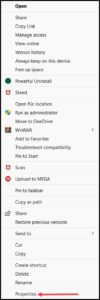The image shows a very blurry, out-of-focus picture of a menu with various selectable options, each accompanied by different icons to their left. The first readable option appears to be "Powerful on Install," marked by a green circle. Below it is an unreadable option with a red badge symbol beside it. Further down, there is an option featuring a badge with alternating yellow and blue symbols. A few positions down, another option is distinguished by a pattern of brown squares. Scrolling three or four options further, next to what seems to be the word "Scan," is the same red badge symbol mentioned earlier. Continuing downwards, there is a red circle with a white dot underneath it, followed by an option two or three positions beyond with black horizontal lines beside what appears to be the word "Share." At the very bottom of the menu rests the word "Properties," highlighted by a red arrow pointing specifically to it. Despite the image's significant blurriness, these details are faintly discernible.